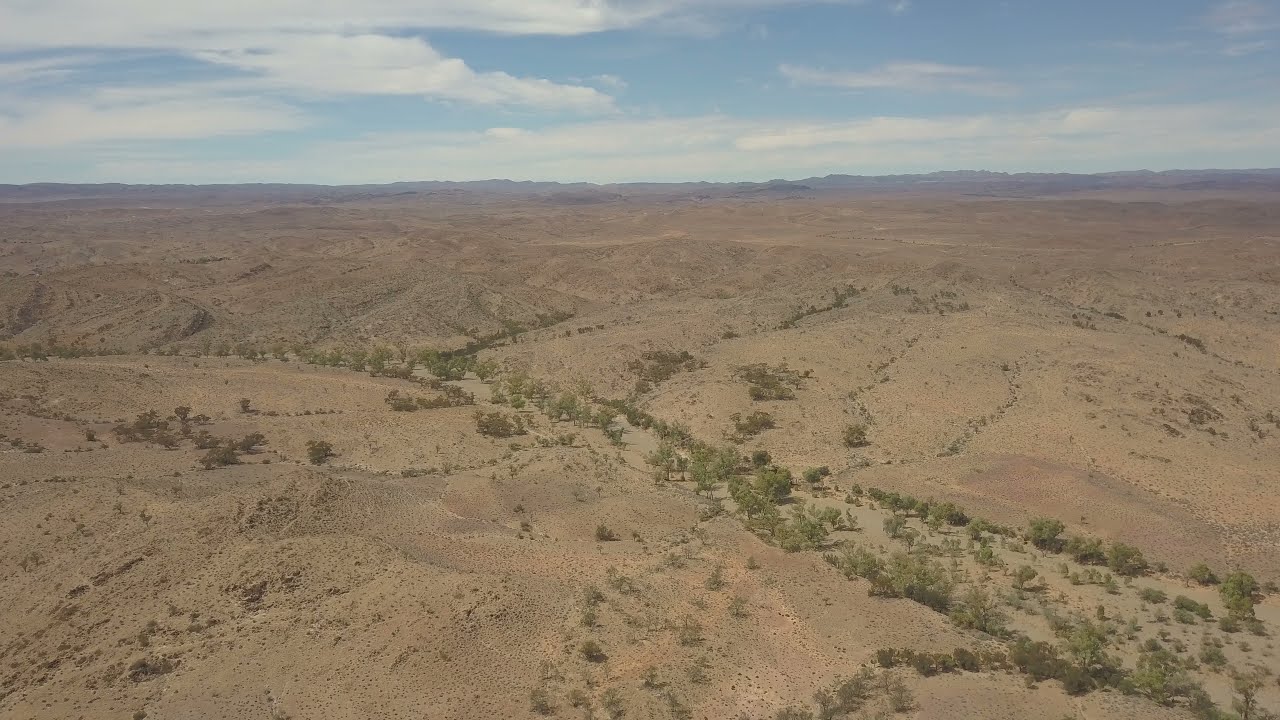This aerial image showcases an expansive, sun-drenched desert landscape. The foreground is dominated by a vast, rolling terrain of tan sand and rocky hills, interspersed with patches of dead grass and sparse green bushes. A winding valley meanders from the middle to the bottom right of the image, lined with small trees and clusters of shrubbery. The arid desert stretches towards the horizon where it meets a distant mountain range, roughly three-fourths up the image. The scene is completed by a clear blue sky adorned with fluffy white clouds, adding depth and contrast to the overall dry and rugged terrain below.